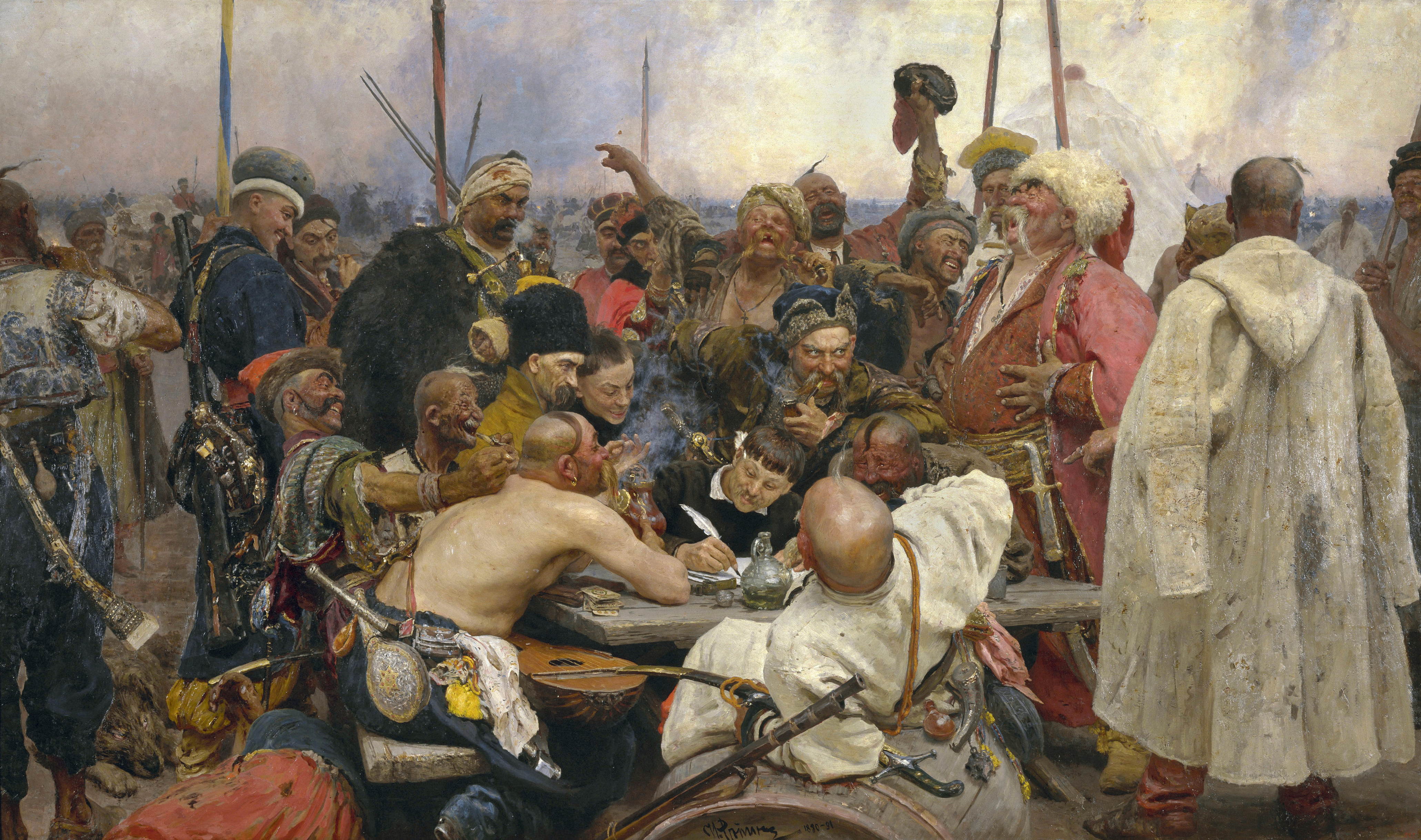This detailed painting depicts a tumultuous scene involving approximately 12 to 15 individuals gathered around a central table. The main focal point is a man in a black tunic with a white undershirt, who is intently signing a piece of paper using a feather quill. Opposite him, another man leans backward, as if reacting to the excitement around him, on a barrel from which a knife and other items are falling. A distinct figure in gold and blue stands behind this man, actively restraining several others. 

In the foreground, near the man in black, is another individual dressed in a brown tunic. He is bald with a noticeable strand of black hair down his face and a brown beard. The crowd in the background consists of various figures displaying a range of emotions; some are shoving, others are smiling or laughing, while a few appear to be arguing. 

Among these individuals, there are men in white tunics with blue accents, brown tunics, pink tunics, and a particularly noticeable man in a dark blue tunic. On the right side of the scene, a prominent character in a pink tunic with a brown undershirt and a frilly white hat is seen laughing heartily. Another man, also standing out due to his long white coat, and another leaning on a barrel, add to the rich, detailed tapestry of this historical tableau.